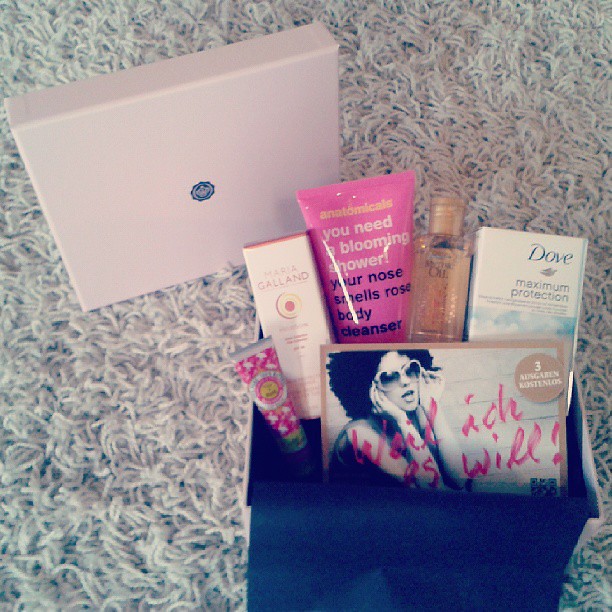In this indoor image, a decorative gift box filled with various personal care products is showcased on a plush, white shag carpet. The box, located in the bottom right of the frame, has an off-white lid adorned with a blue company logo positioned in the top left. Inside the open box, there's an assortment of items including a pink bottle labeled "You Need a Blooming Shower, Your Nose Smells Rose" body cleanser, Dove Maximum Protection soap, body oil, and what looks to be a CD cover featuring a woman with puffy hair and sunglasses. The array of colors within the box includes white, off-white, blue, pink, yellow, gray, and tan, enhancing the aesthetic appeal of this potential gift set.